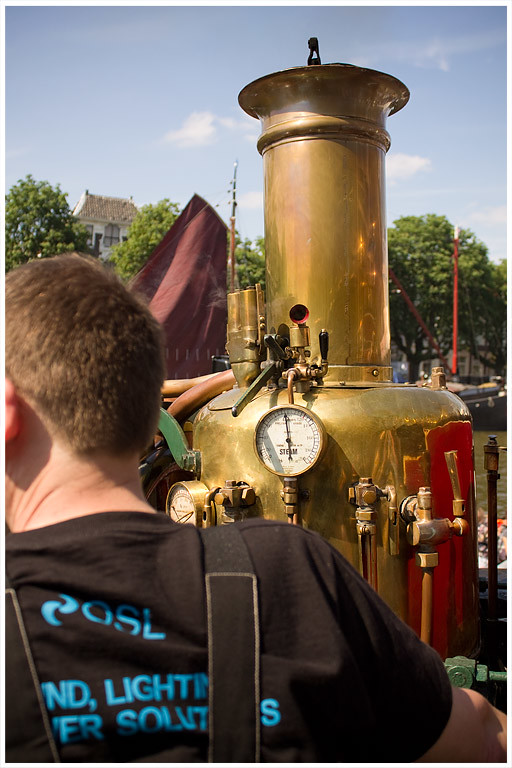The photograph, taken outdoors on a clear, sunny day, features a vintage steam machine or high-pressure apparatus prominently displayed against a backdrop of tree canopies. This intricate device, shimmering in gold or brass metal, consists of a wide cylindrical tank topped with a tall, narrower chimney-like structure. The machine brims with antiquated elegance, adorned with multiple valves and a conspicuous round pressure gauge that hints at its purpose as a steam boiler.

Front and center in the image stands a man with his back to the camera. He sports a black t-shirt with light blue text, potentially indicating an OSL logo along with the words "lighting" and "solutions." His short, light brown hair is closely cropped, and suspenders or backpack straps drape over his shoulders.

The scene, set in what appears to be a park with lush green trees, evokes a sense of warm weather, likely during summertime, underscoring the machine’s status as a historical relic rather than an operational device.